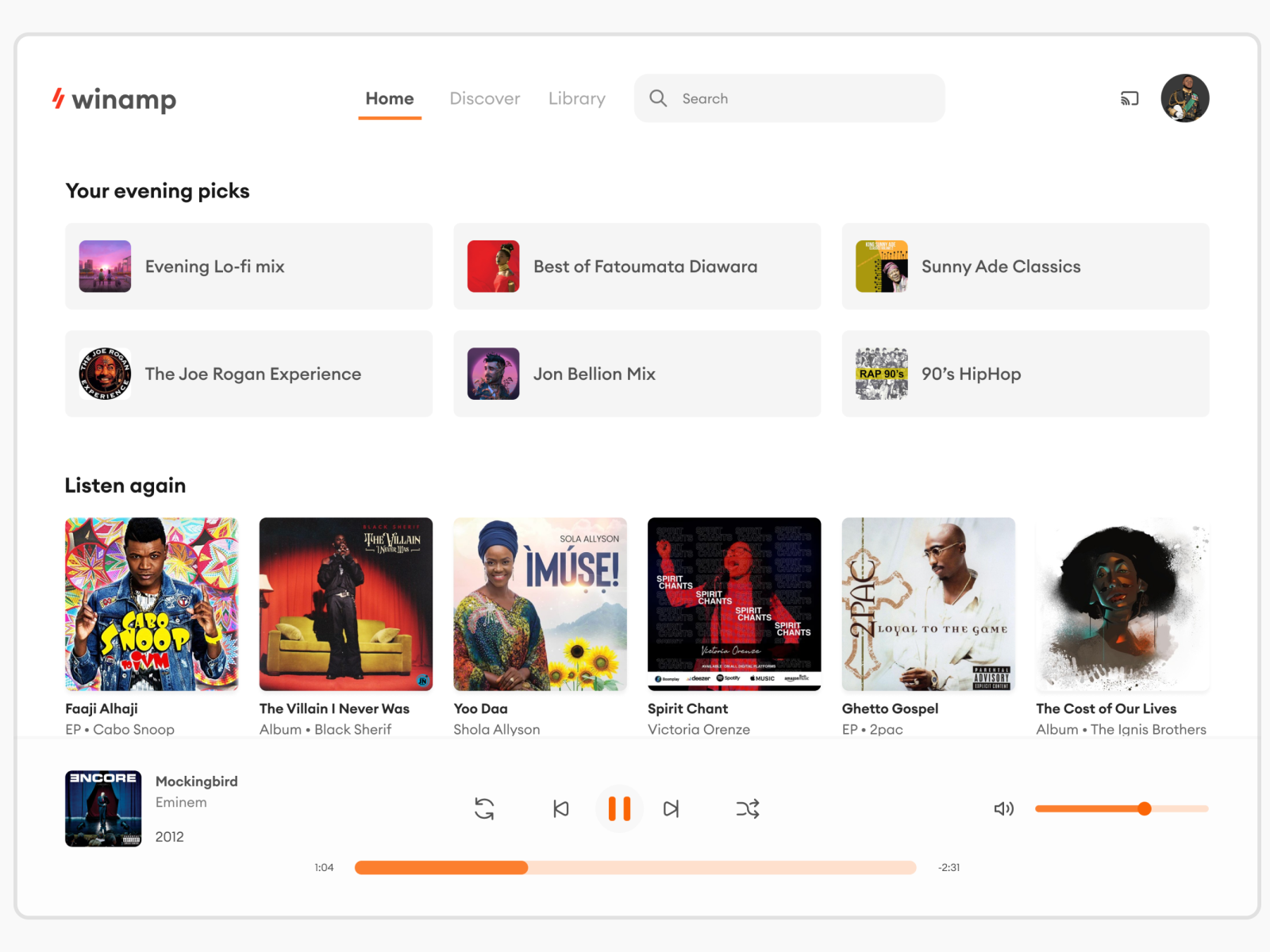A screenshot from Winamp's user interface displays a sleek, modern design dominated by black and orange hues. At the top, a navigation bar includes options such as 'Home,' 'Discover,' 'Library,' and a gray search bar for easy access. An icon on the upper right side depicts a white silhouette of a person against a dark background, while 'Home' is underlined in orange, indicating the current section.

Prominently featured is a section labeled "Your Evening Picks," showcasing various playlists and podcasts including "Evening Lo-Fi Mix," "The Joe Rogan Experience," "Best of Fort Jomato," "John Bellen Mix," "Sonny Aide Classics," and "90s Hip Hop." Each entry is accompanied by a relevant image, presumably album covers or podcast thumbnails.

Below, the "Listen Again" section invites users to revisit recently played tracks or albums, displaying six distinct covers with corresponding artist images. Highlights include albums from Fadji Eladji, 'The Villain I Never Was,' Yudonna's 'Spirit Chante,' 'Ghetto Gospel,' and 'The Cost of Our Lives.'

Further down, a track titled "Mockingbird" from the album 'Encore' is in the playback queue, evidenced by the album cover and an orange progress bar that is approximately a quarter complete. A pause button is prominently displayed, with a volume control on the right showing the sound level slightly more than halfway up.